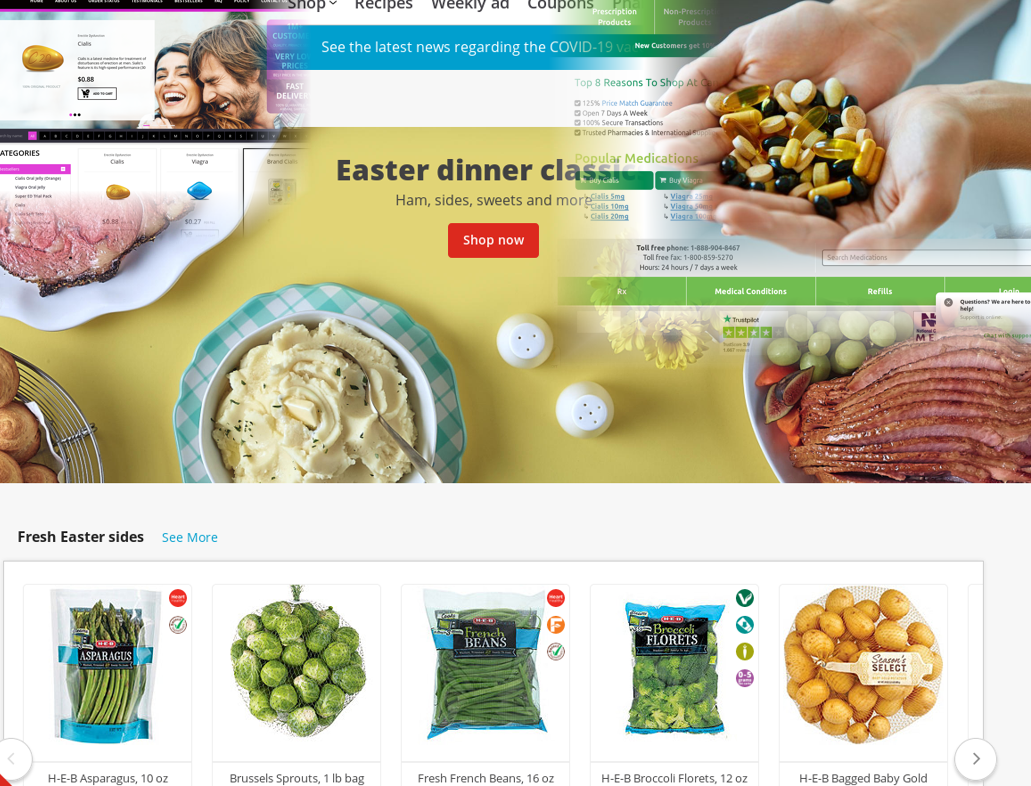This image appears to be from a grocery store's website, but it's complicated by an overlapping image of medications that creates some confusion. At the top of the website, there is a navigation bar with sections labeled "Shop," which has a drop-down arrow, followed by "Recipes," "Weekly," "Add," "Coupons," and more, although the rest is blurry. 

The banner at the top has an image overlay issue, presenting two different visuals. In the background, there's a picture of a hand holding various pills with the text "Popular Medications," suggesting that medication purchasing might be a feature of the website. However, in the foreground, there is a clear grocery-themed setup. This part shows a promotional message reading "Ham, Sides, Sweets, and More" with a red "Shop Now" button written in white. 

The foreground banner image depicts a neatly set table featuring two white salt and pepper shakers, small yellow flowers, cold meats with grapes, a fig, a white bowl containing something yellow, a small bowl of mashed potatoes with a silver spoon, a metal wire container holding what looks like scones, and a white plate with more meat. Below this banner, the website highlights "Fresh Easter Sides," offering options such as asparagus, brussel sprouts, fresh French beans, H-E-B broccoli florets, H-E-B bagged baby gold potatoes. 

The composition of this image is quite intricate and somewhat confusing due to the overlaid pictures, blending elements of grocery shopping with pharmaceutical supplies.